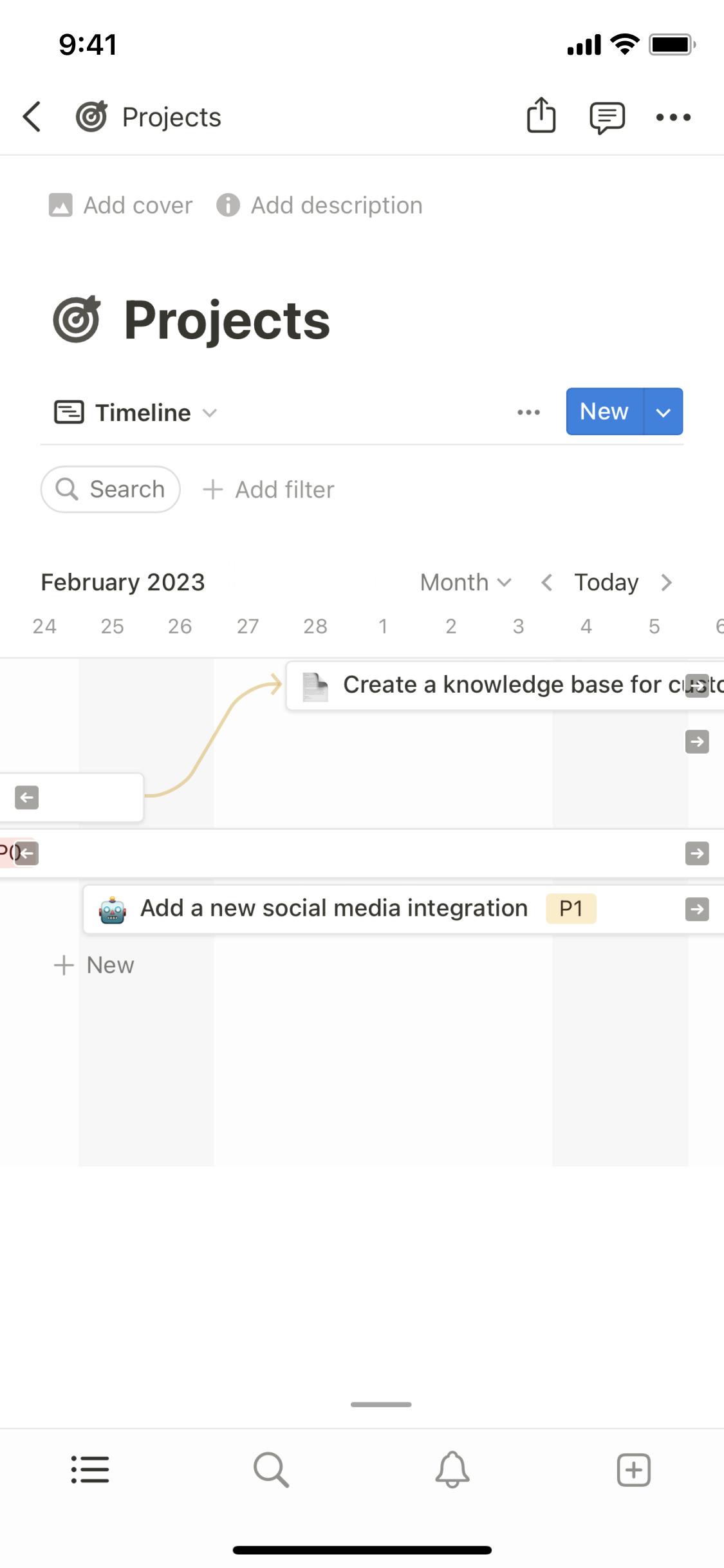This vertically oriented rectangle image, likely a screenshot from a cell phone, features a detailed display of a project management application. At the very top left corner, it shows the time "9:41" in black text. On the top right corner, icons indicate full cell phone signal with four bars, a full Wi-Fi signal, and a fully charged battery.

The background of the image is entirely white. Directly below the time, a left-pointing arrow and a target symbol are displayed. Next to these symbols, the word "Projects" appears. Moving towards the right, there are icons for sending, captioning, and an options menu indicated by three horizontal dots. This section is divided by a thin gray line.

Further down, there are options to "Add Cover" and "Add Description." In bold print, accompanied by an icon, the word "Projects" appears again alongside a target symbol. Below that, "Timeline" is written with a dropdown menu next to it. On the far right, there are three horizontal dots followed by a blue box labeled "New" with a white downward arrow. This section is also separated by a thin gray line.

Next, a search bar encapsulated in an oblong box and a "Plus Filter" button are visible. As you continue to scroll down, there's a date function displaying "February 2023" with a dropdown menu, and today's date is highlighted.